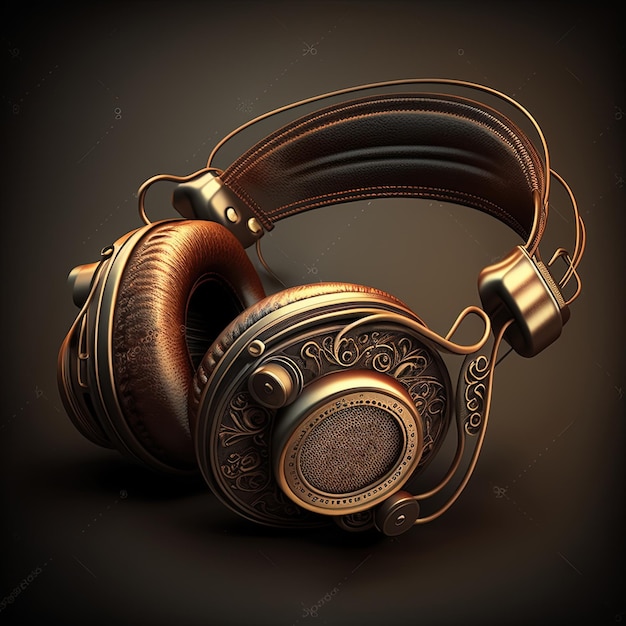A pair of vintage steampunk-inspired headphones is captured against a black background with crisscrossing, translucent, spiderweb-like lines and dots. The headphones are a detailed 3D rendering, featuring an antique aesthetic with a predominantly brown, copper-like color palette. Both the earmuffs and the headband are crafted from a leather-like material, showcasing intricate, ornate designs that evoke a sense of Victorian England or a pirate-esque vibe. The brown ear coverings are accompanied by speaker-like elements on the outer earmuff areas, and the entire set is artistically aged yet maintains a polished finish. The image offers a zoomed-in view, highlighting the craftsmanship and the gleaming, well-preserved state of these old-fashioned yet distinctly unique headphones.